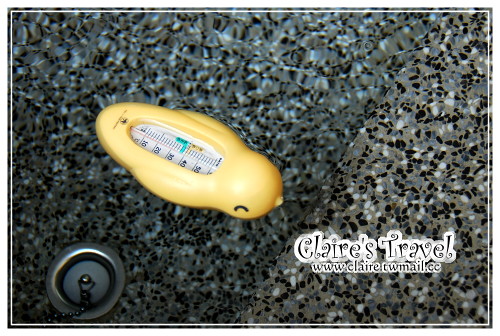This detailed photo captures a downward view of a surface with a black, white, and grayish-blue granite marble appearance. In the bottom right corner, the surface bears the text "Claire's Travel, www.claire.twmail.cc." On the table sits a distinctive yellow duck thermometer; the thermometer is enclosed within a plastic yellow duck casing. The display on the duck shows a temperature reading of approximately 50 degrees, highlighted by a blue area. Below the duck on the left, there is a round metal object featuring a central round metal ball. This ball is connected by a chain comprised of small linked balls, which together form a string attaching to the central metal ball on the round metal object.